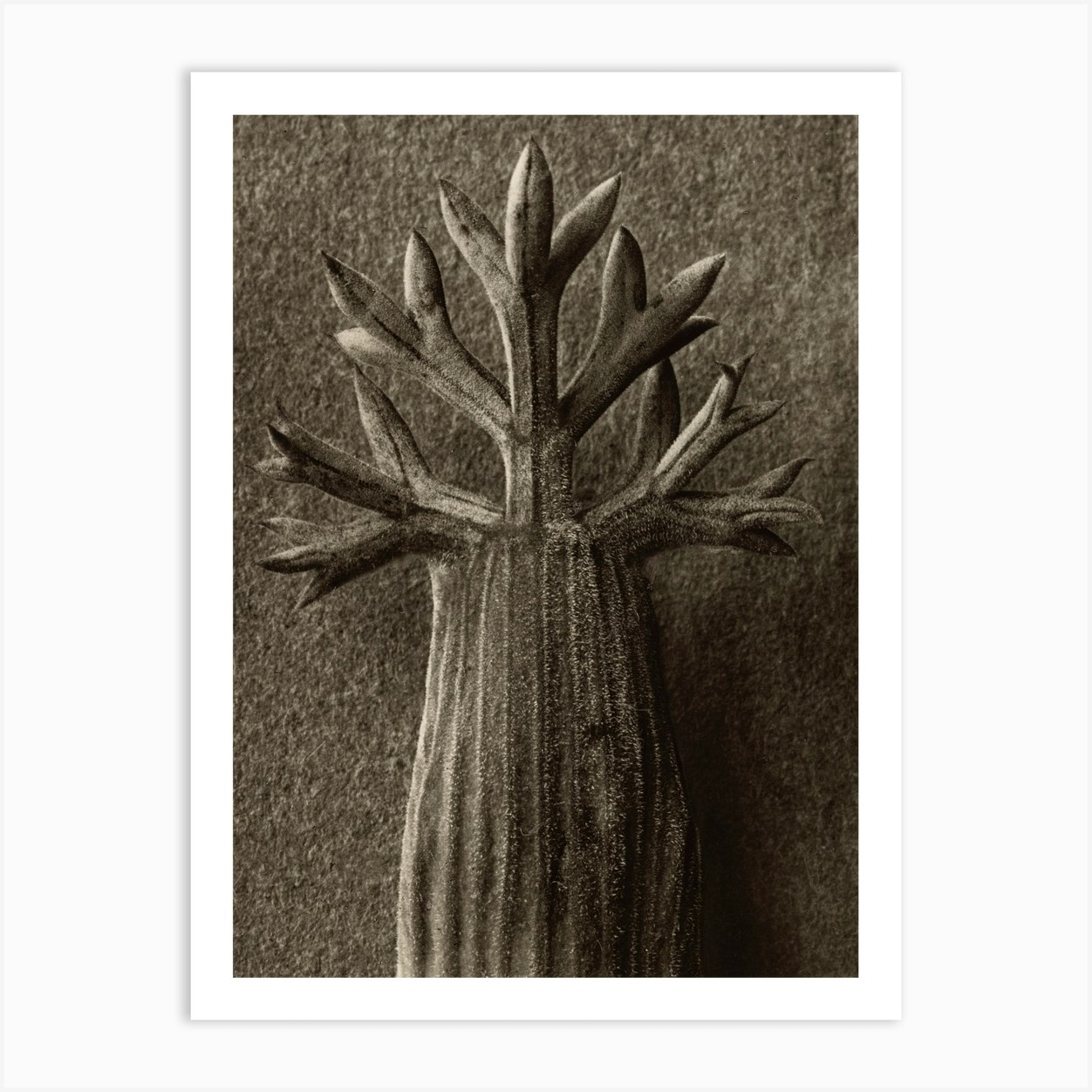The image is an art print featuring a central object that resembles an abstract, iron-made plant or cactus, positioned vertically from the bottom middle to the top. The composition is rendered in shades of black, white, and gray, giving it a monochromatic, almost sepia tone. The plant-like figure has a thick base and consists of three main branches, each with additional offshoots, the central one being the tallest. The background of the image appears grainy or textured, akin to sand, and the entire print is encased in a white border, framed against what seems to be a white wall. The object itself has a velvety appearance with intricate lines and patterns, described as looking like leaves and chicken feet. The print is balanced and could either be a highly abstract photograph, possibly AI-generated, or a depiction of a 3D model or plush toy mimicking the form of a cactus.